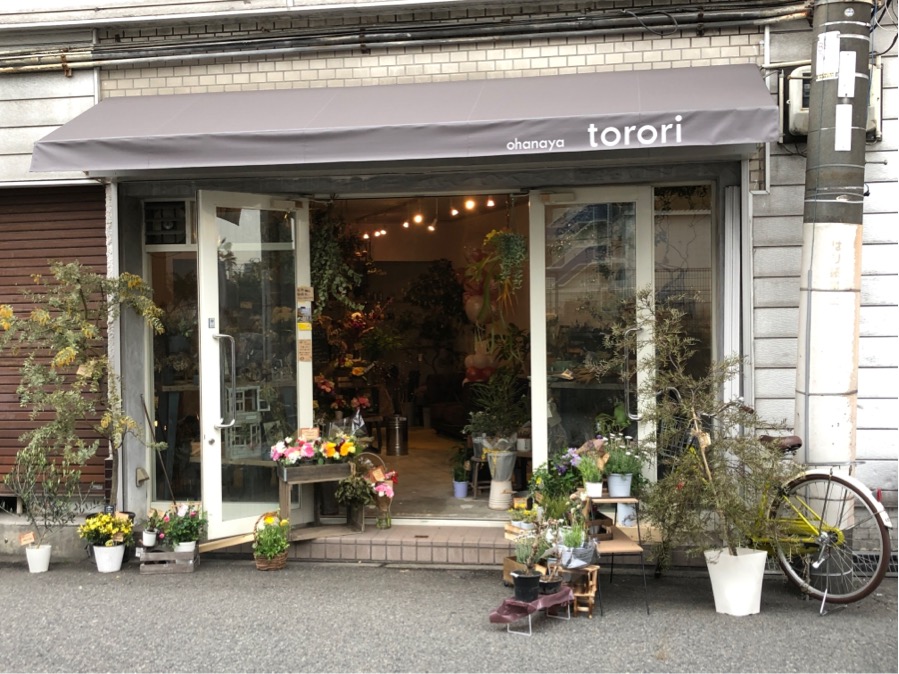This photograph depicts the charming exterior of a florist's storefront. The storefront features prominently white-framed glass doors, thrown open to welcome visitors, and tall glass windows that flanking the entrance. The doors provide a peek inside, revealing an abundance of vibrant plants and flowers arranged in various vases and containers.

The building exterior combines different textures, with the left side appearing as brown wood, the right as white wood, and the top as tan brick. A notable black awning, emblazoned with the name "Ohanaya Torori" (with varying interpretations of the exact lettering), extends over the entrance.

In front of the shop, the ground is pebbled cement with a small brick step leading up to the doors, adorned with a delightful array of tiny planters filled with colorful blooms, cascading down onto the street. A white pot holds a small tree, positioned in front of a quaint bicycle parked nearby. This charming, floral haven exudes a welcoming, verdant allure, inviting passersby to explore the botanical beauty within.